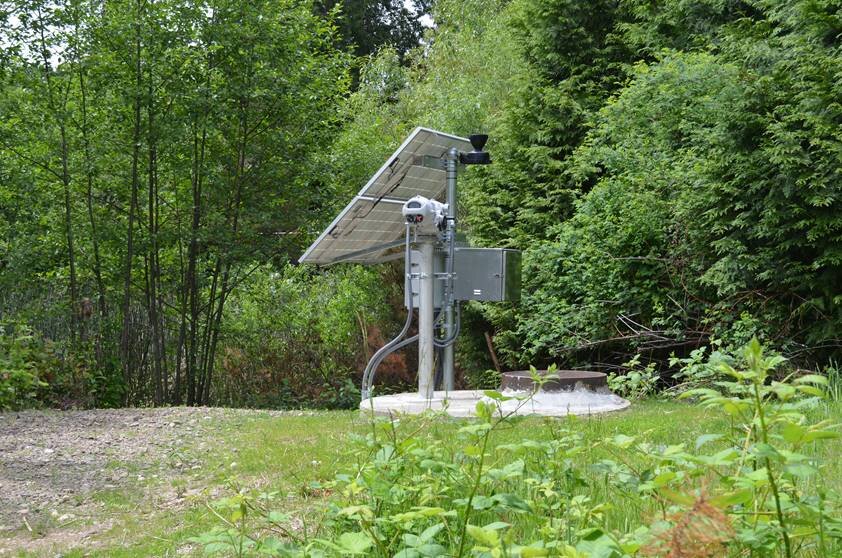The daytime photograph captures a secluded solar panel station situated on the outskirts of a wooded area. Dominated by tall, lush green trees, wild weeds, and tiny white flowers, the surroundings are teeming with greenery. The solar panel, angled to maximize sunlight absorption, is fairly large, approximately four by three feet, and features a grid-like, white surface. The structure includes a tall, metallic pole anchored into a circular concrete slab. Attached to the back of the panel are several components, including long wires and a protruding silver box, likely housing the control mechanisms. A small gravel road meanders through the site, providing access to the unit amidst the vibrant natural landscape.